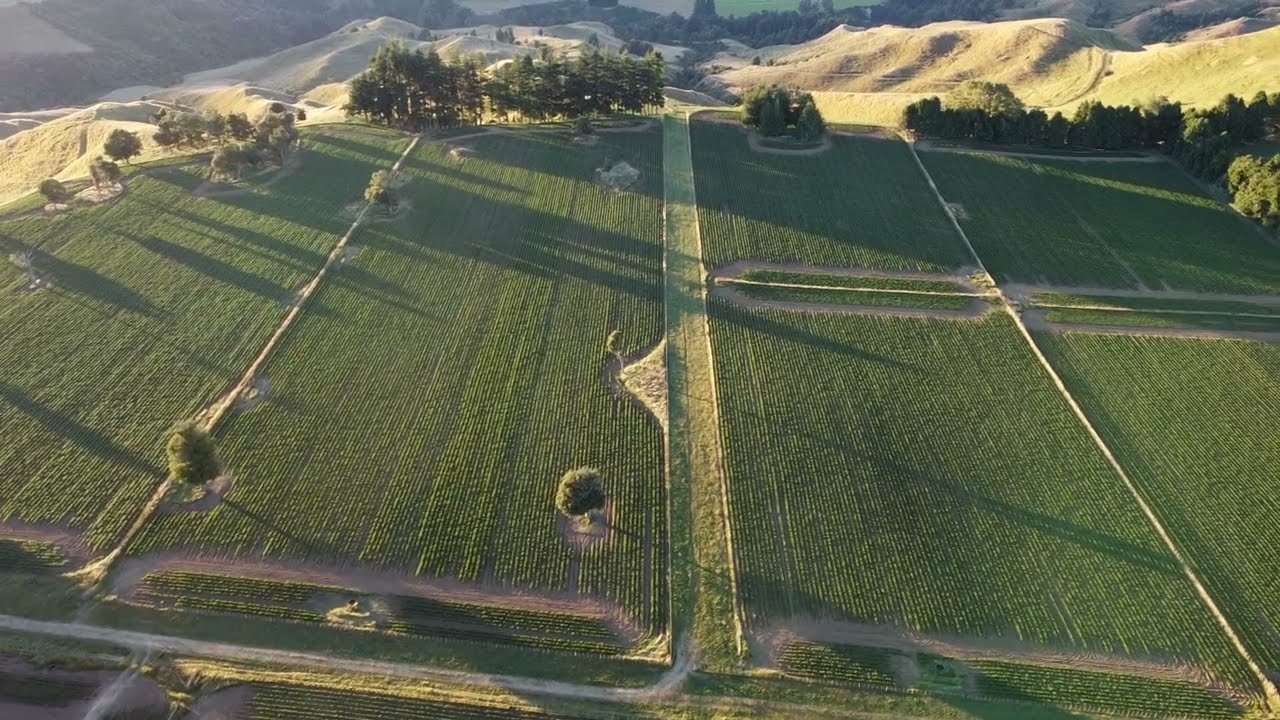The image depicts a large, predominantly green field, likely used for farmland, captured from an aerial perspective around sunrise or sunset, as indicated by the long shadows cast by the sparse trees in the background. The field appears meticulously landscaped with several clearly defined pathways and plots, suggesting active cultivation or preparation for future development. The land is organized into four equal square lots on the right and two elongated rectangular lots on the left, all rich with green grass. There are no visible people, vehicles, or buildings, highlighting the field's remote and undeveloped nature. In the background, gently rolling hills or low mountains create a natural boundary, adding to the scene's rural ambiance. The primary colors of the image are various shades of green, mixed with some grayish tones, illustrating a well-maintained agricultural or undeveloped area.